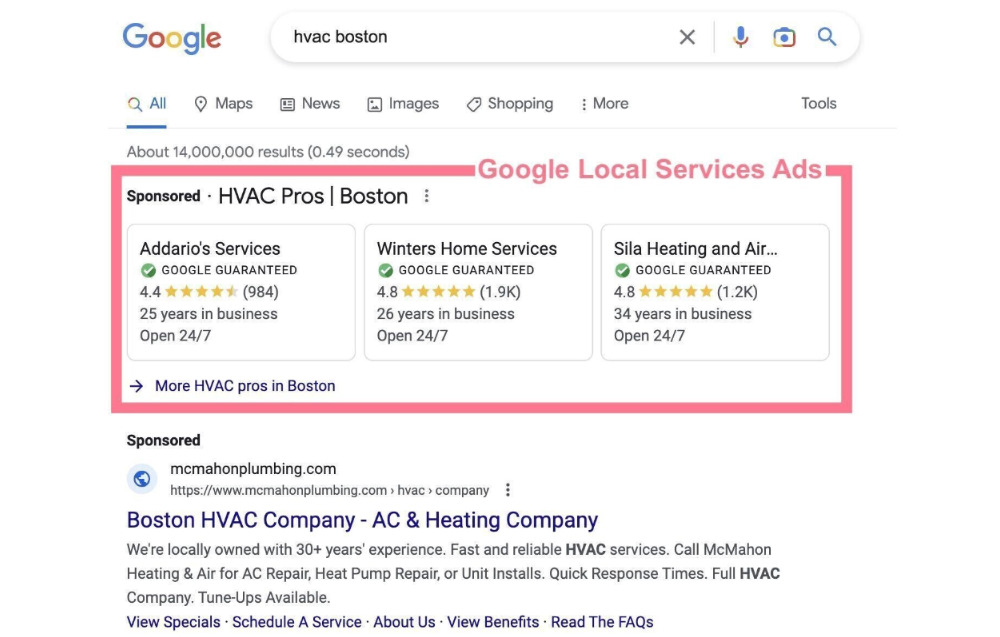The image depicts a Google search results page for the query "HVAC Boston." The screenshot highlights a section dedicated to Google Local Services Ads positioned at the top of the page. This highlighted section prominently features three sponsored listings:

1. **Adareo Services** - Rated 4.4 stars.
2. **Winters Home Services** - Rated 4.8 stars.
3. **Sila Heating and Air** - Rated 4.8 stars (name is partially cut off).

Each of these listings includes high user ratings, indicative of their quality. Additionally, a separate sponsored result is displayed below this section, labeled as "Boston HVAC Company, AC and Heating Company," from mcmanplumbing.com. The focus of the highlight appears to be on the top three sponsored ads, possibly due to their prominence and high ratings, while the logic behind the exclusion of the lower sponsored result remains unclear. The overall search results emphasize top-rated HVAC service providers in the Boston area.